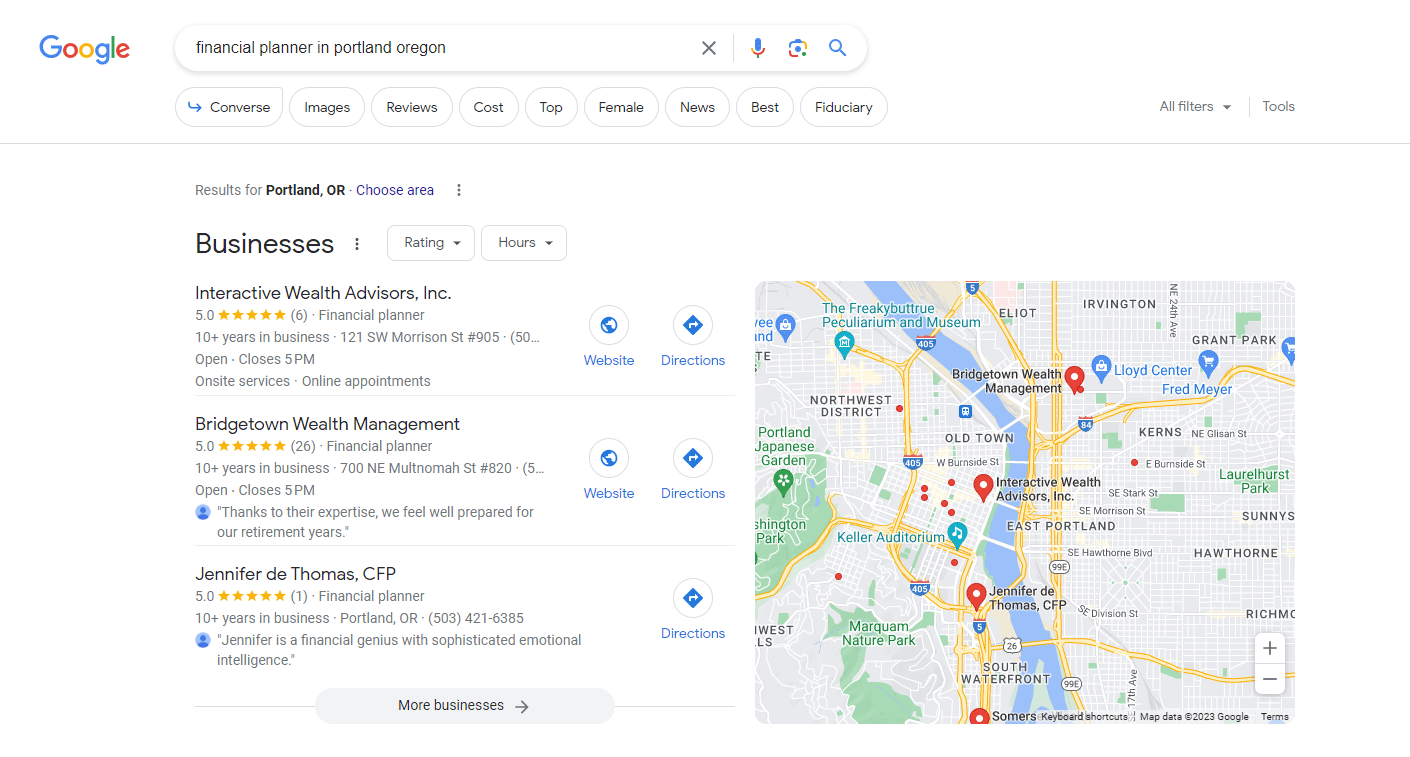The image shows a Google search page with the keywords "financial planner in Portland, Oregon" entered in the search bar. Just below the search bar are various clickable tabs, including "Converse," "Images," "Reviews," "Cost," "Top," "Female," "News," "Best," and "Judiciary." The search results highlight three top financial planning businesses in Portland, Oregon. 

1. **Interactive Wealth Advisors**:
   - Over 10 years in business
   - Offers on-site services and online appointments 
   - Address displayed
   - Closes at 5 PM

2. **Bridgetown Wealth Management**:
   - Also with over 10 years in business
   - Defines itself as a financial planner
   - Address displayed
   - Closes at 5 PM
   - Praised for their expertise, preparing clients well for retirement

3. **Jennifer D Thomas, CFP**:
   - Over 10 years in business
   - Located in Portland, Oregon
   - Described as a financial genius with sophisticated emotional intelligence

All three businesses are rated five stars. To the right, there is a map showcasing the locations of these businesses in Portland, making it easier for users to visualize where each one is situated.